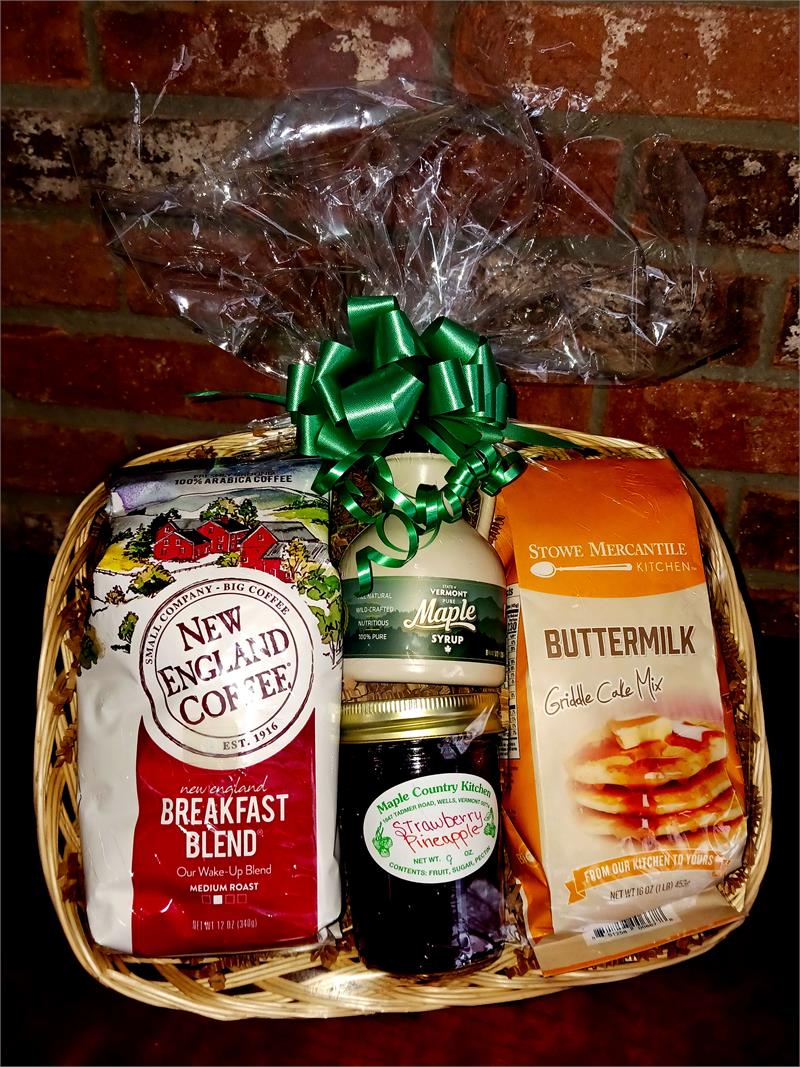The image depicts a festive holiday gift basket elegantly wrapped in cellophane and adorned with a beautiful green bow at the top. The basket itself is a charming brown woven design, positioned against an old, dark red brick wall that adds a rustic touch. Inside the basket, to the left, there is a bag of New England Coffee's Breakfast Blend. On the right side, lies a bag of Stowe Mercantile Kitchen Buttermilk Griddle Cake Mix. Centrally nestled between these items is a homemade-style jar of strawberry pineapple preserves. Above the preserves, you'll find an old-fashioned jug containing Vermont maple syrup. The entire arrangement is neatly displayed, lying on what appears to be a brown table, and the photograph, taken at night with a flash, emphasizes the neatness and illumination of the gift items, contrasting against the worn, historic brick backdrop.